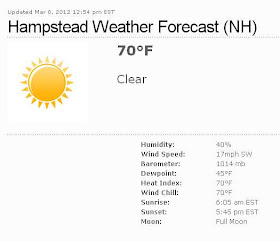The image depicts a detailed weather forecast for Hampstead, New Hampshire. It features a light gray or off-white square layout. At the very top left corner, in small print, it indicates the update time as March 8th, 2012, at 12:54 p.m. EST. Below that, in bold black letters, it reads "Hampstead Weather Forecast (NH)".

On the left side, a small white square showcases a bright yellow sun symbol, indicating sunny weather. To the right, the temperature is displayed prominently in bold black text as "70°F". Directly underneath, the weather condition is noted as "Clear".

A gray line separates the temperature section from additional weather details listed on the right side in black type. These details include:
- Humidity: 40%
- Wind Speed: 17 mph southwest
- Barometer: 1014 mb
- Dew Point: 45°F
- Heat Index: 70°F
- Wind Chill: 70°F
- Sunrise: 6:05 a.m. EST
- Sunset: 5:45 p.m. EST
- Moon Phase: Full Moon